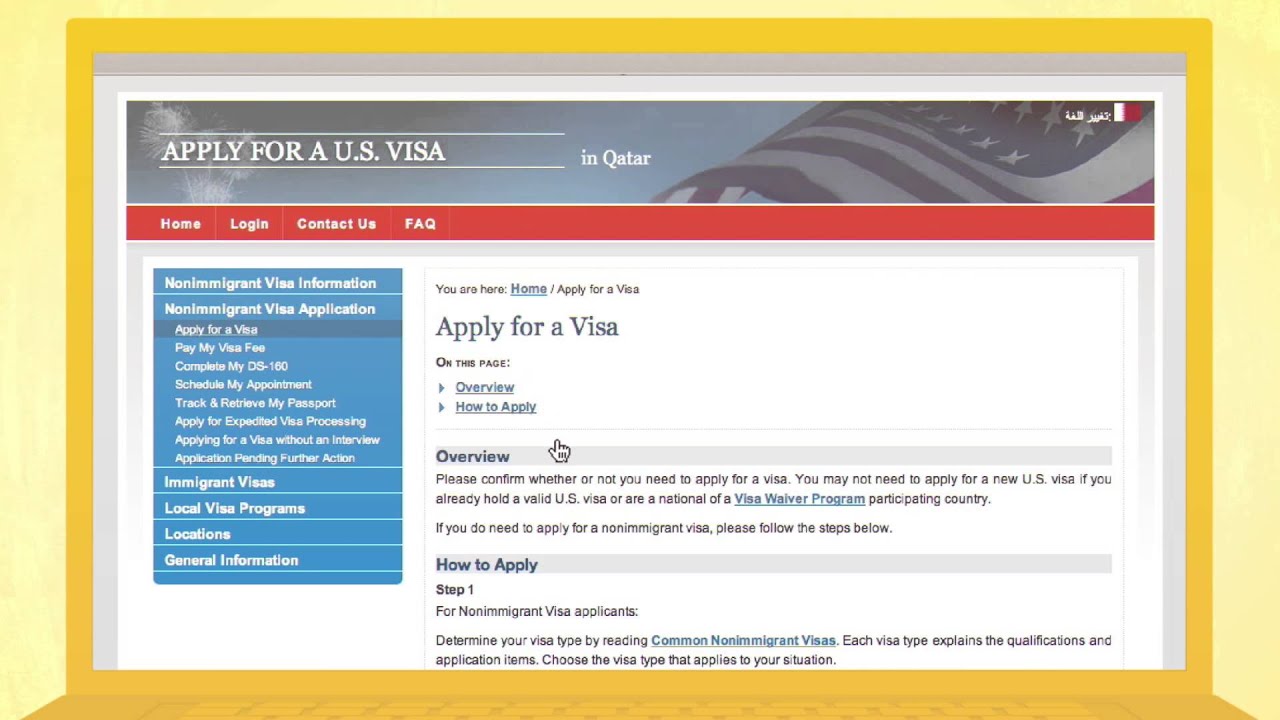**Detailed Caption**:

This image appears to be a screenshot of a website intended for applying for a USA visa from Qatar. The interface is in landscape orientation with a distinctive, layered border design. The outermost border is a light yellow, while an inner segment running along the bottom edge transitions to a darker, more orange-yellow tone, creating an additional boundary within the original border. 

At the top of the page, a thin gray banner stretches across, followed by a lighter gray banner that continues horizontally and down the sides. Beneath these banners lies the main content area, distinguished by another gray banner at its upper part.

The central section features a partially unfurled American flag on the right, alongside possible iconography like Qatar's flag on the upper right. Prominently displayed in this area are the words "Apply for a USA Visa in Qatar" on the right side of the banner. Below this, a red banner is positioned for emphasis.

On the left side of the main content area, there is a blue box with selectable options. The option "Apply for a Visa" is highlighted. The right side of this blue box contains detailed instructions in white for the visa application process. Below these instructions, there are clickable links, including an "Overview" button and a "How to Apply" button.

Further down, the website provides a detailed breakdown of the application process. Under headers like "Overview" and "How to Apply," which are set against gray bars, step-by-step instructions and text guides (referred to here as "tests") are presented, beginning with "Step One" and continuing with subsequent steps.

This structured layout and design elements make the user experience both clear and navigable for anyone seeking to apply for a USA visa from Qatar.